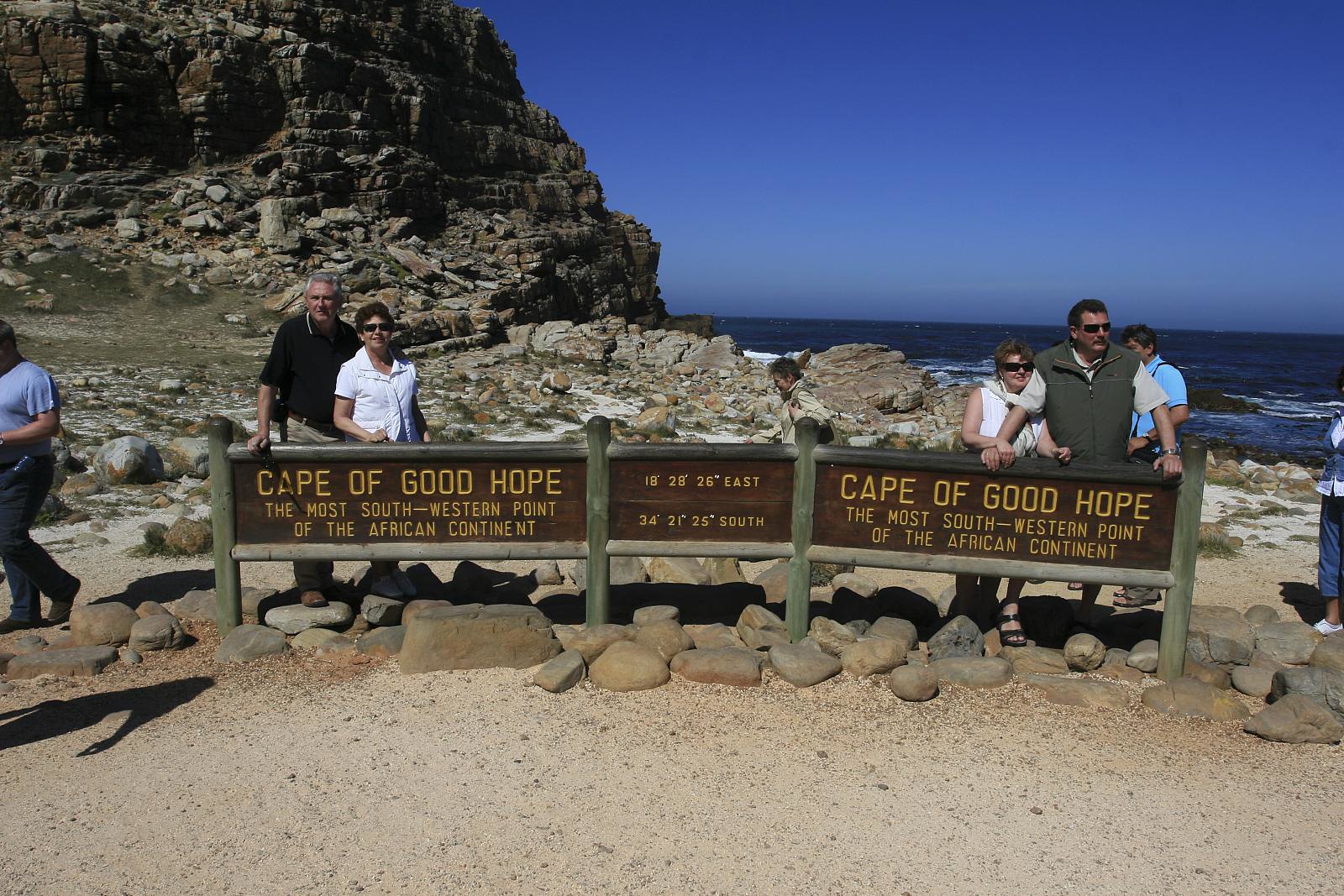This captivating photograph captures a picturesque tourist spot at the Cape of Good Hope, the most southwestern point of the African continent. The focal point of the image is a prominent wooden sign with brown and yellow lettering, framed by green logs, which reads: "Cape of Good Hope, the most southwestern point of the African continent," along with latitude and longitude coordinates. In the foreground, jagged brown rocks and a sandy walking path lead to the sign, while the midground is bustling with tourists.

Two couples, both consisting of a man and a woman, are posing to the left and right of the sign, all wearing sunglasses and exuding a relaxed, vacation vibe. The left couple is positioned closer to the rocky hillside, while the right couple is set against the stunning backdrop of a vast, blue ocean. Additional visitors, who appear to be mostly white, are scattered along the sandy path and rocky terrain, mingling or taking in the breathtaking views.

In the background, the scenery features a rugged shoreline with white caps visible on the ocean waves, and the distant horizon meets a clear, cloudless blue sky. This serene yet vibrant scene encapsulates the natural beauty and tourist allure of the Cape of Good Hope.